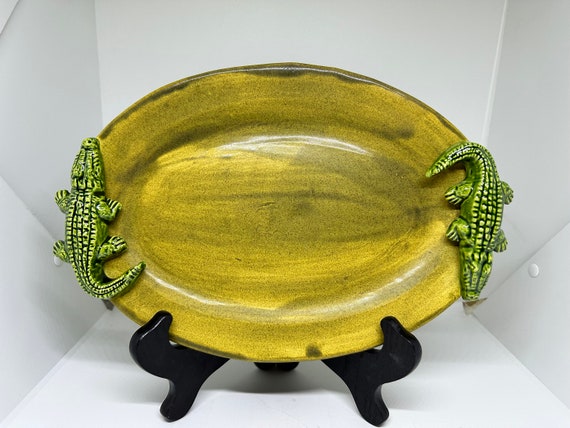The image showcases a realistic-style photograph of a vintage, gold-colored, oval-shaped ceramic plate, displayed in a white, cubby hole-like miniature stage. The plate sits upright on a black, three-legged wooden stand, centrally placed to highlight its details. The ceramic plate features two alligators or crocodiles in light green and yellow hues, with reptilian scales prominently depicted. The alligator on the left is facing up, while the one on the right is facing down. The plate has an aged appearance, with a base coat of yellow paint accentuated by brown and black smears to create an antiqued effect. The overall background is the interior of the white box, enhancing the plate's display and making it a focal point for viewers.